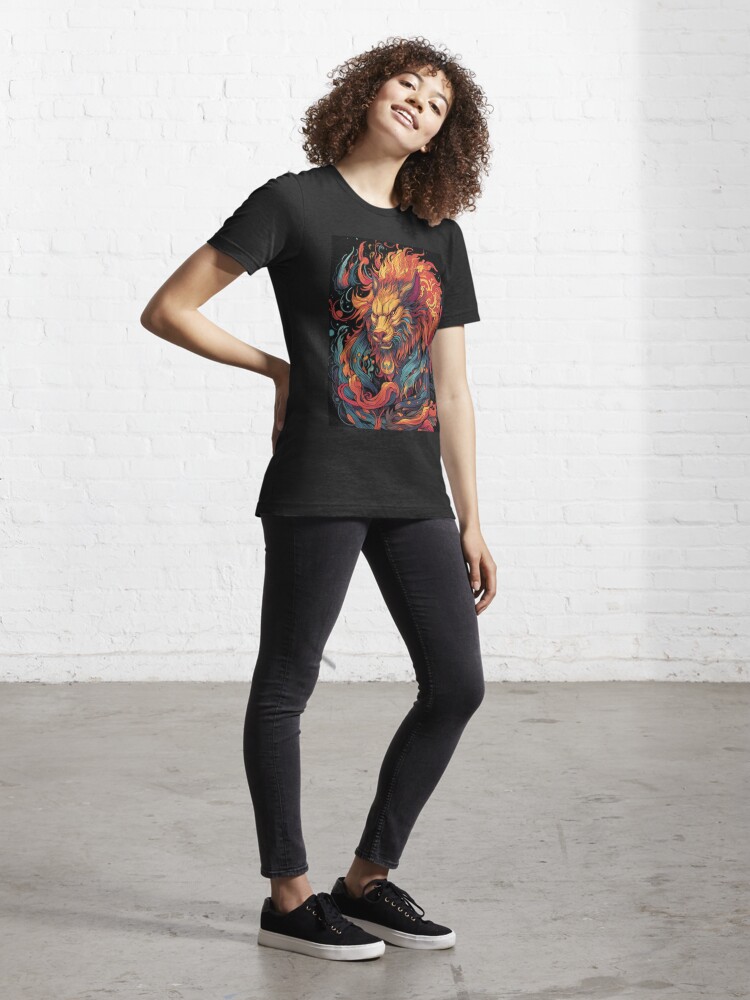In the photograph, a young woman stands confidently in the center of a room with white-painted brick walls and a gray concrete floor, suggesting a potential setting for a clothing store magazine. She has shoulder-length, tight-knit curly brown hair and a light brown complexion. Her head is tilted back, to the left, and slightly upward, with a subtle smile gracing her lips. Her right hand rests on her hip while her left arm hangs naturally by her side. She is wearing a black t-shirt adorned with a large, cartoony yet dramatic graphic of a lion in vibrant orange, accented with turquoise and red hues. The design of the lion takes up a significant portion of the shirt, possibly reminiscent of an iconic movie character. She pairs the t-shirt with tight black skinny jeans and completes her outfit with black laced-up sneakers that feature a white rubber sole, resembling a Vans style.